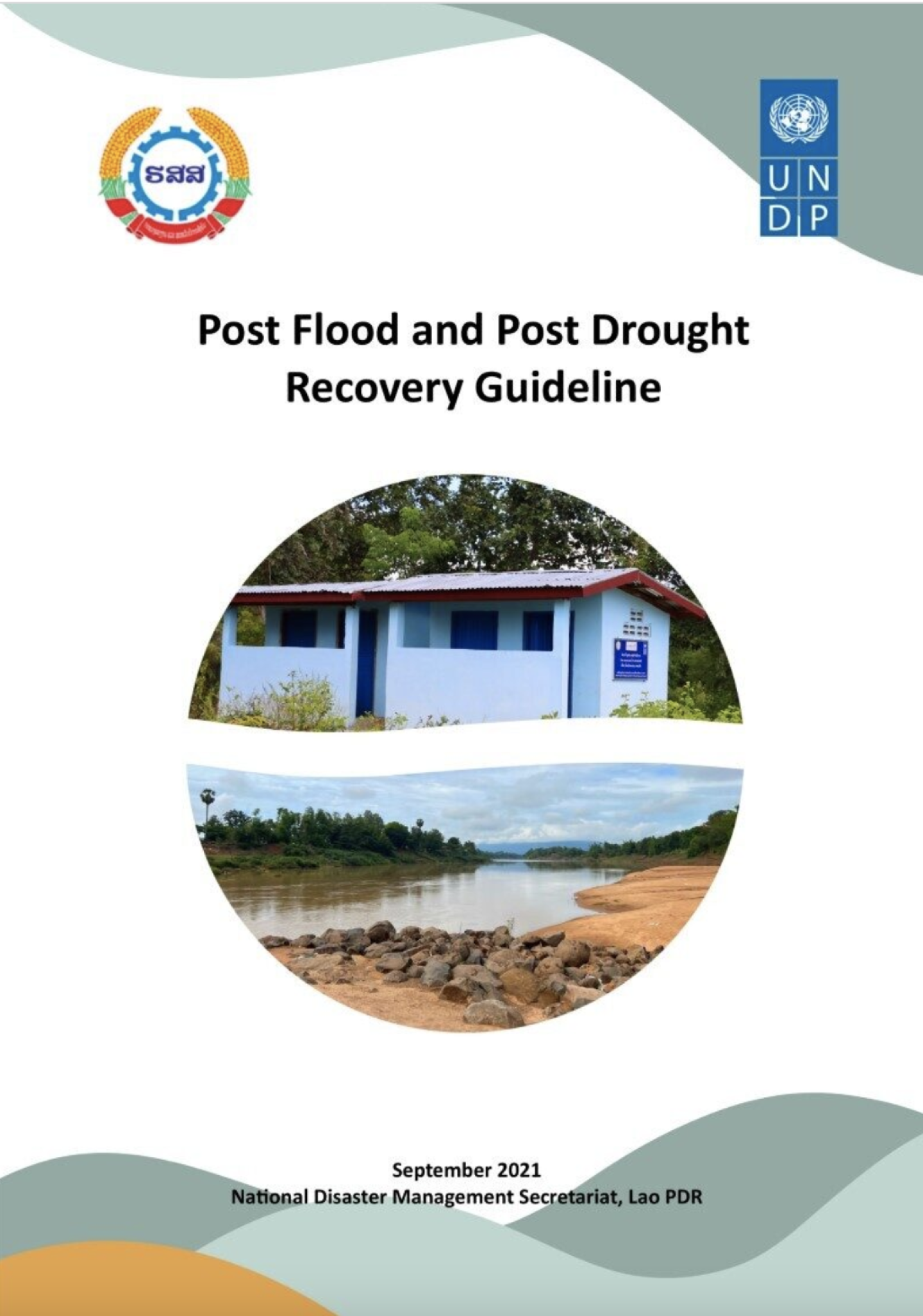The promotional cover image for the "Post-Flood and Post-Drought Recovery Guideline" by the United Nations Development Programme (UNDP) features a white background with decorative swirly patterns in grayish-green at the top and bottom edges. In the upper right-hand corner, there is a blue box with the UNDP logo. The upper left-hand corner displays a circular logo with intricate details: a blue gear center enclosed by a ribbon-like design, featuring yellow tips resembling corn, transitioning to red and green hues around the perimeter.

Centrally, the title "Post-Flood and Post-Drought Recovery Guideline" is prominently displayed. Below the title, there is a round, bisected photograph. The upper half showcases a small, blue building with a red roof, surrounded by trees, suggesting a flood-affected area. The lower half presents an image of a muddy, low-water riverbed, bordered by rocks and sparse vegetation, depicting a drought-affected zone. The absence of people and animals in the images emphasizes the environmental focus.

At the bottom of the image, textual information reads "September 2021 National Disaster Management Secretariat, Lao PDR," indicating the publication date and relevant organization in Laos.